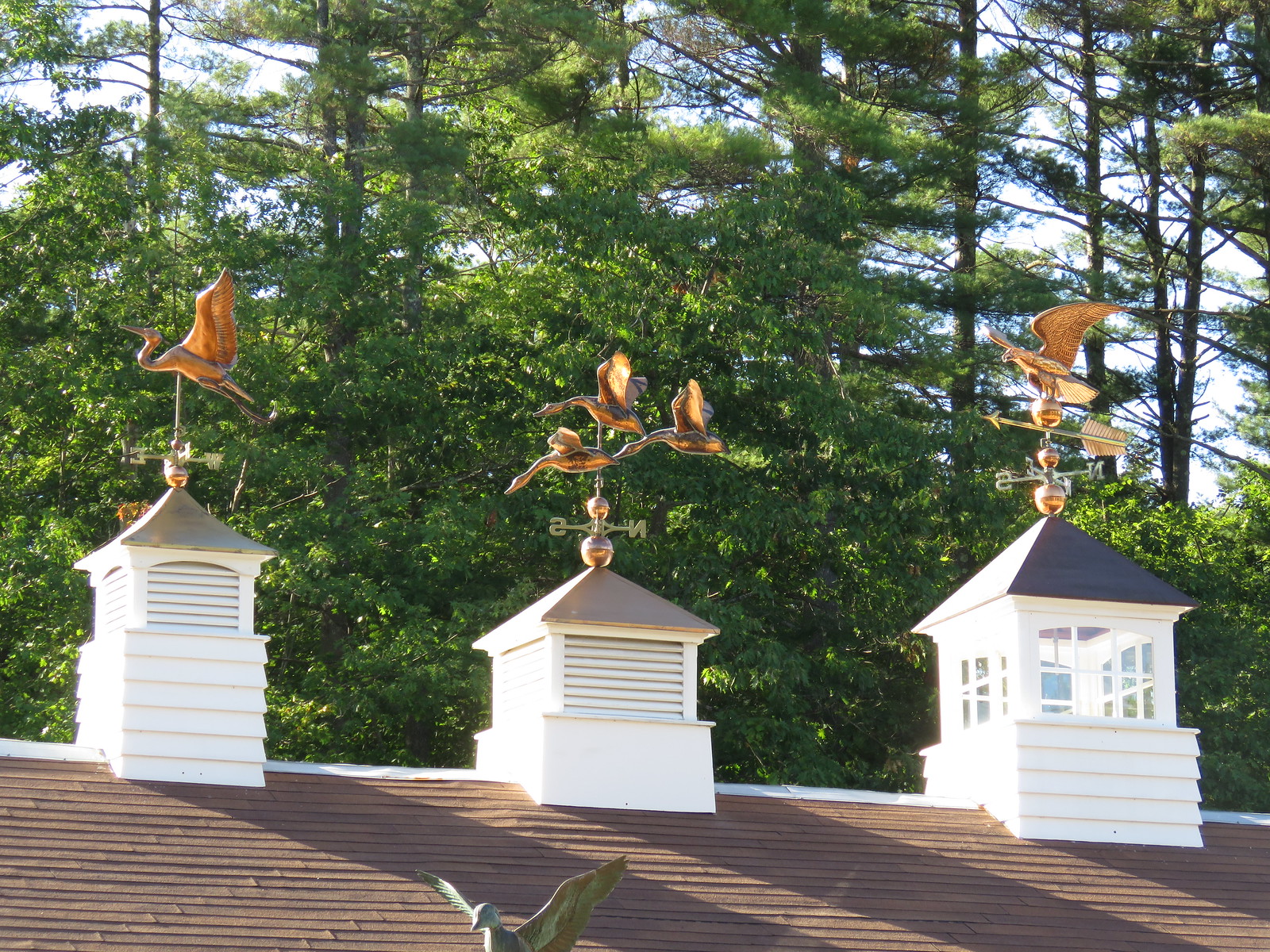This color photograph, horizontally oriented, captures the intricate scene atop a pitched brown roof, set against a backdrop of towering dark green pine trees. Three miniature white structures, resembling tiny houses with pointed gray roofs and small windows, sit atop the roof. The structure on the left features louvers for windows and is adorned with a decorative seabird that resembles a heron. The middle structure, smaller in size, is topped with a set of three golden geese sculptures, all arranged in a flying formation, serving as a weather vane to indicate wind direction. The largest structure on the right has traditional windows and is crowned with a striking American eagle, wings spread, serving a similar weather vane function. In the foreground of the image, perched on another roof, is a small bird, accentuating the New England architectural style of the scene. The entire composition showcases a vivid interplay of functional and decorative elements, set against the lush, natural backdrop.